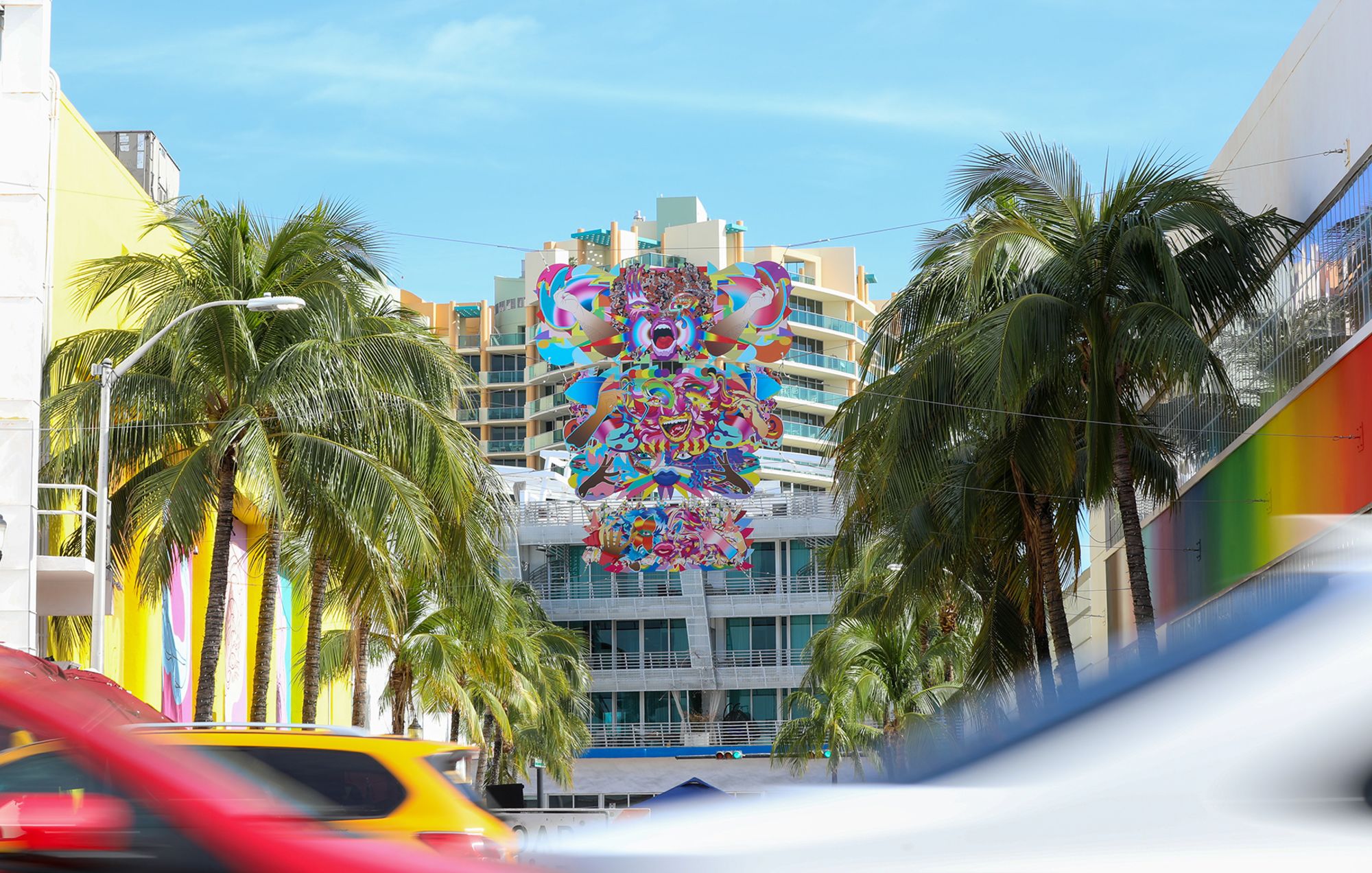The image captures a vibrant, tropical scene in a parking lot and street setting, likely in a southern region. Framed by tall palm trees on either side, the street stretches toward a substantial, multi-story white hotel building in the background. The sky is a brilliant blue with scattered clouds, enhancing the vivid atmosphere. Along the street, there are brightly colored buildings in hues of yellow, lemon, aqua, pink, purple, and more, accented by a bright yellow car and a fire-engine-red vehicle near the hotel. There are streetlights, windows, and a little balcony visible. The hotel in the background showcases a striking mural or art piece featuring carnival-like creatures in vibrant colors such as purples, greens, blues, reds, and yellows, seemingly strung up with strings like a large, decorative banner. The overall scene is bathed in ample sunlight, making every detail clear and lively.